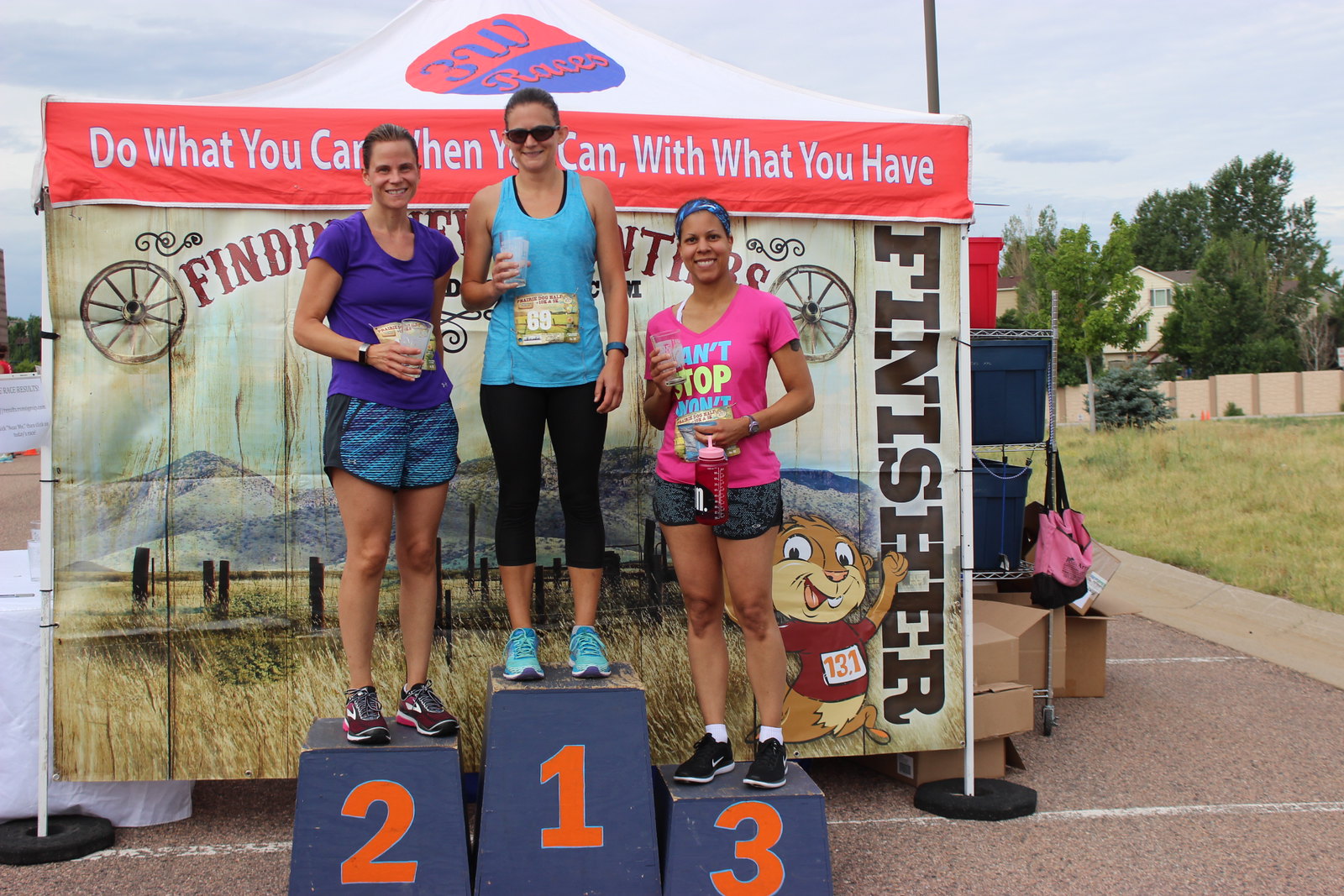In this vibrant outdoor scene, three women proudly stand on a blue finisher's podium, labeled with large orange numbers 2, 1, and 3, signifying their respective rankings in a recent race. The woman in the middle on the number 1 spot stands the tallest, wearing a light blue tank top, black leggings, blue sneakers, and sunglasses, displaying her race bib number 69. She holds a cup in her hand and beams with a triumphant smile. To her right, on the number 2 podium, a woman in a purple Under Armour-style shirt and bluish-purple running shorts holds a cup, her race bib partially obscured. On the left, the number 3 finisher wears a pink t-shirt with gray running shorts and a blue bandana, holding a water bottle and smiling broadly. Behind them, a tent features a banner with red and blue lettering, stating, "Do what you can when you can with what you have," alongside a playful cartoon chipmunk or groundhog and additional wording that reads "3W Races." The grassy area and a parking lot dot the background under a clear, blue sky, completing this joyous post-race moment.